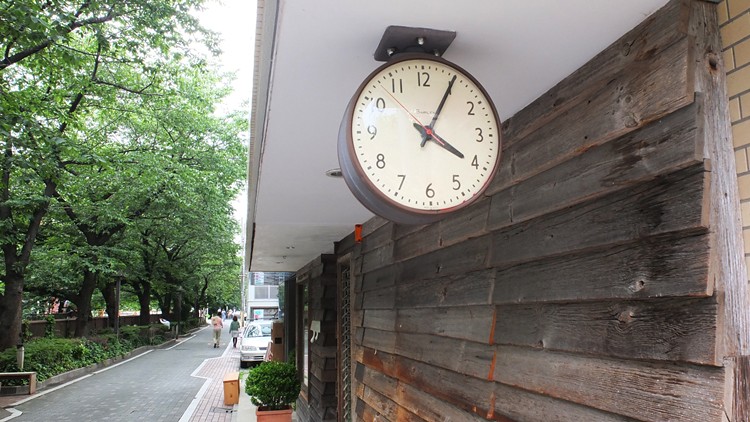This photograph captures a detailed streetscape scene. To the left of the image, there is a gray brick road lined with a white stripe, which transitions to a brown and red brick road leading up to a wood-clad storefront. The wooden facade of the building, weathered to a gray-brown hue, is complemented by a small terracotta planter with a dark green bush. Adjacent to the building is a white car parked facing forward. Two individuals are visible walking down the road, one dressed in a red shirt and khaki pants, while the other wears a blue shirt paired with a skirt of indeterminate color. 

Above the wood-paneling, and extending from the building’s roof overhang, hangs a prominent large clock with a white face and black hands indicating the time as 4:05, with the second hand nearing the 11. The outer frame of the clock is a dark brown. Visible in the top right corner of the image are tan or light brown bricks forming part of the building’s structure behind the wooden panels. The scene is backdropped by a line of fully green trees and an overcast sky, adding to the tranquil ambiance.